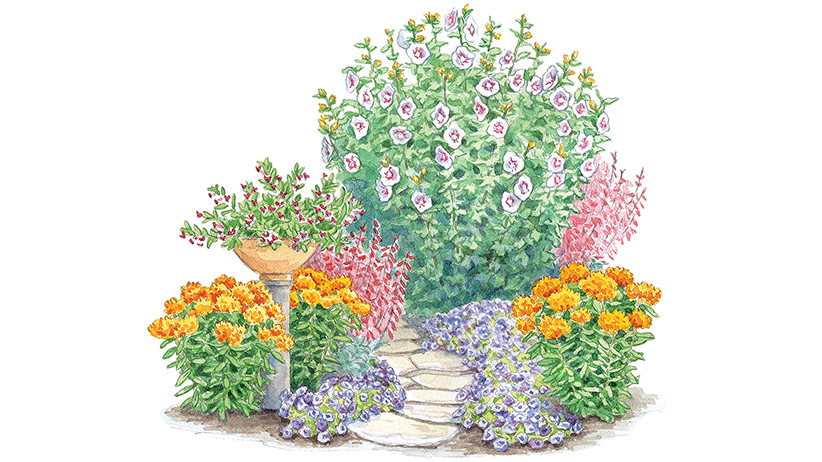This detailed artist's sketch depicts a vibrant corner of a garden, meticulously recreated with colored pencils. Central to the composition is a stone pathway composed of various shaped beige-gray riverstones, flanked by a plethora of blooming flora. Lining the base of the path are clusters of low-lying purple flowers. These are bordered by longer-stemmed golden-orange flowers, which in turn are complemented by towering vertical pinkish-red blossoms. To the left of the path, a stone bird bath with a gray pillar holds a bowl of tiny deep-red, heart-shaped flowers. Further along the path, the vegetation obscures its end, taking the viewer's eye to a larger bush with white flowers accented by purple centers and unopened yellow buds. The drawing showcases an array of textures, with shaded brown ground suggesting dirt or mulch beneath the flora. The background remains completely white, focusing attention on the garden scene, devoid of human presence.